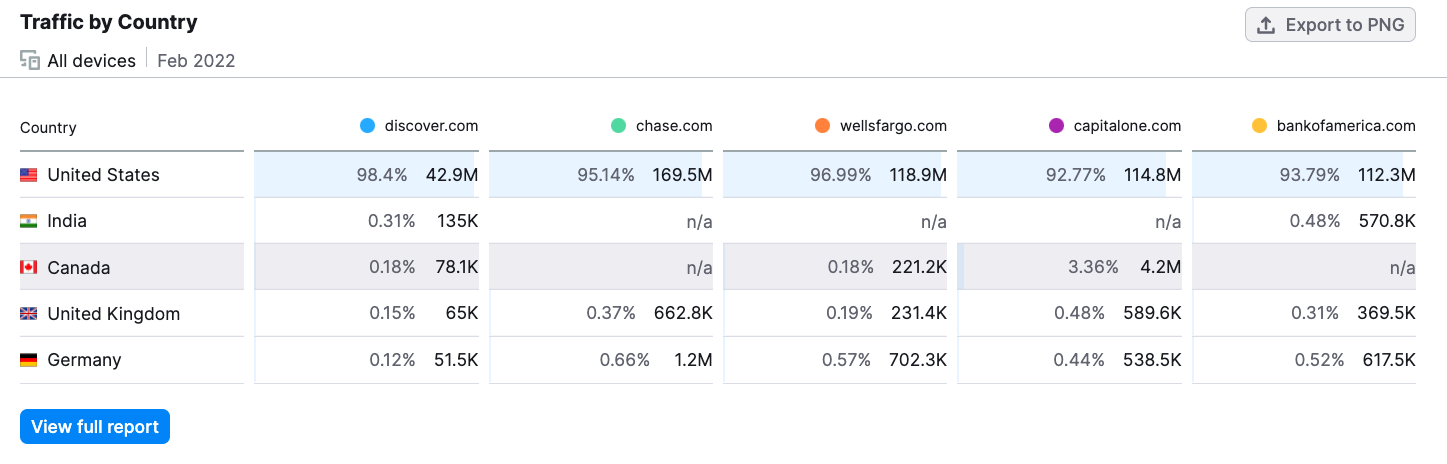The image is a detailed screenshot of several charts positioned in the top-left corner, titled "Traffic by Country". Directly beneath this title, the data is categorized under "All Devices February 2022". In the upper-right corner of the screenshot, there is a button labeled "Export to PNG," allowing users to download the charts.

At the top of the charts, the United States is the leading country, with its data extending horizontally across various sections, each representing a different website: Discover.com, Chase.com, Wells Fargo, Capital One, and Bank of America. The chart also includes data for other countries: India, Canada, United Kingdom, and Germany.

For the website Chase.com, both India and Canada have "N.A." marked in their respective sections. Similarly, India shows "N.A." for Wells Fargo and Capital One, while Canada has "N.A." for Bank of America. All other fields are populated with both a percentage and what appears to be a monetary amount.

In the bottom-left corner of the screenshot, a button labeled "View Full Report" is visible, likely providing more in-depth information when clicked.